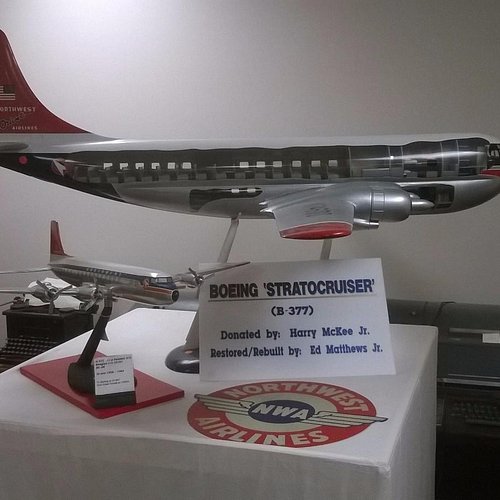The image features a detailed display showcasing two model airplanes. The main focus is a realistically crafted model of the Boeing Stratocruiser B-377, positioned from left to right on a table. This model, a reflective silver with multiple windows, red wingtips, and an American flag at the tail, represents the historic Northwest Airlines. It's accompanied by a placard noting its donation by Harry McKee Jr. and restoration by Ed Matthews Jr. Nearby, a second, smaller model of a Stratocruiser stands on a red platform supported by a black arm. While its accompanying information sheet is difficult to read, the display is enriched with a red and white Northwest Airlines insignia, featuring the NWA symbol flanked by airman wings. In the background, another plane's nose points towards the camera, adding depth to the exhibit, which is further accentuated by an adjacent old-fashioned typewriter, collectively creating a nostalgic assortment of aviation memorabilia.